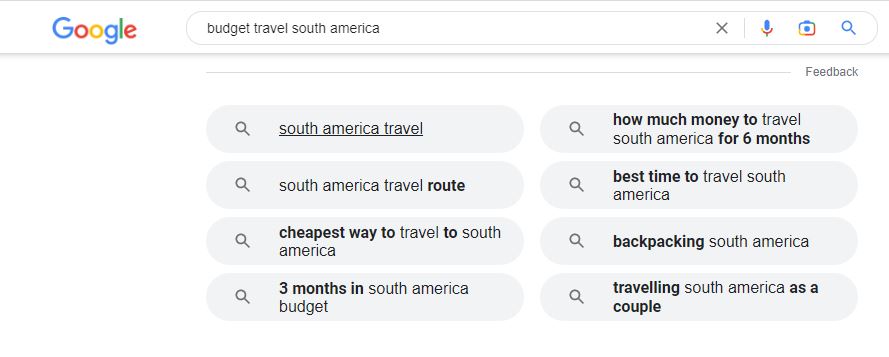This screenshot captures Google search results displayed on a clean, white background. At the top of the frame, a thin light gray line stretches horizontally across the entire width. The header, positioned beneath this line, begins with the multicolored Google logo on the left and is followed by an elongated, pill-shaped search box with a light gray outline. Inside this text box, black search terms appear on the left, while the far right features four icons: a dark gray 'X', a multicolored microphone, a multicolored camera, and a blue magnifying glass. A thin vertical light gray line separates the 'X' from the other icons.

Below the header is a medium gray shadow overlaying the body of the page, and a light gray line centers on the page beside the light gray text "Feedback." Beneath this, the page displays four rows, each containing two pill-shaped buttons with a light gray outline. Each button has a dark gray magnifying glass icon on the left, followed by search suggestions in text. 

The search suggestions include:
1. Underlined: "South America travel."
2. Bolded and not bolded: "How much money to travel South America for six months."
3. Partially bolded: "South America travel route."
4. Bolded and not bolded: "Best time to travel South America."
5. Partially bolded: "Cheapest way to travel to South America."
6. Partially bolded: "Backpacking South America."

This detailed breakdown showcases the elements and layout of a Google search results page in a clean and organized manner.